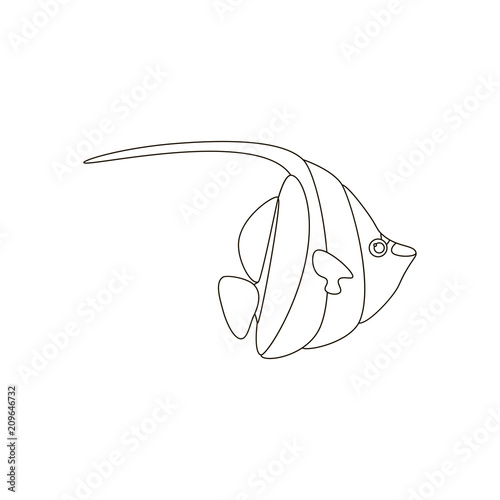The image features a simple, computer-generated graphic of a fish, depicted in a pen-and-ink style. It appears to be a black-and-white outline without any color, situated against a plain background. The fish is drawn from a side view, with a distinctly pointed nose and a small round eye. Its body is shaped similarly to that of an angelfish, exhibiting a triangular form. The fin on top of the fish is notably long and curves to the left, while the other fins stick out from the sides, giving the impression that one can see through the fish's body. 

Positioned in the center of the image, the graphic itself is uncluttered and lacks intricate details, showing only curvy lines to illustrate the fish's contours. This straightforward design suggests it could be used for various purposes, such as a kid's coloring book or a stock photo on a website. A watermark reading "Adobe Stock" encompasses the entirety of the image, with additional text in the lower left corner stating "Adobe Stock number 209-646-732," arranged vertically. Despite the simplicity of the sketch, these elements combine to create an abstract yet recognizable depiction of a fish.